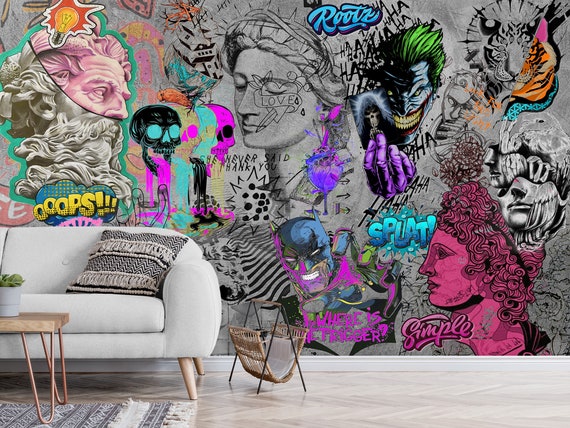In this image, a modern living room is depicted, featuring a cushy and comfortable white sofa adorned with black and white throw pillows and complemented by a light wood coffee table positioned in front of it. On the side of the sofa, there’s a stylish u-shaped wooden magazine rack with black legs. The floor is a tan-colored laminate or hardwood, with white wooden baseboards along the walls adding a touch of elegance. 

Dominating the scene is a large, vibrant mural on the gray wall behind the sofa. This mural, resembling graffiti art, showcases a blend of historical and contemporary figures. The centerpiece includes abstract depictions of Greek statues, including a Greek goddess and a male torso. Nearby, the notorious Joker from Batman is vividly illustrated with a blue face, green hair, red cheek scars, and purple gloves. 

Below the Joker, Batman is depicted wearing a cape, characterized by a determined expression. The mural also features various other faces, both black and purple skulls, and bursts of abstract elements such as hearts. Interwoven within this eclectic imagery are distinct words like "oops," "roots," "splat," "simple," and "where is trigger," rendered in purple, blue, and pink, adding layers of intrigue and visual interest to the artwork.

A small planter with green leaves adds a fresh touch to the coffee table, enhancing the modern yet eclectic aesthetic of the room. The contrast between the sophisticated furnishings and the vibrant, dynamic mural creates a unique and visually stimulating living space.